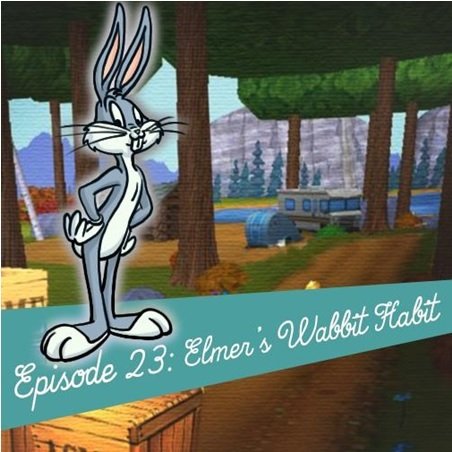This image appears to be a title card from a Bugs Bunny cartoon episode titled "Episode 23, Elmer's Wabbit Habit." Bugs Bunny stands confidently with his hands on his hips atop a green banner featuring the episode title in white cursive letters. The background is set in a colorful cartoon campsite, complete with a Winnebago, a tent, a log cabin, and large stones or mountainous areas. Tall trees border the scene, though the leaves are depicted in a low-poly style, reminiscent of video game graphics. The foreground includes dirt roads, shipping crates, and a few bushes, one of which is red. The overall image is brightly lit and clearly detailed, presenting a lively and engaging animated scene.